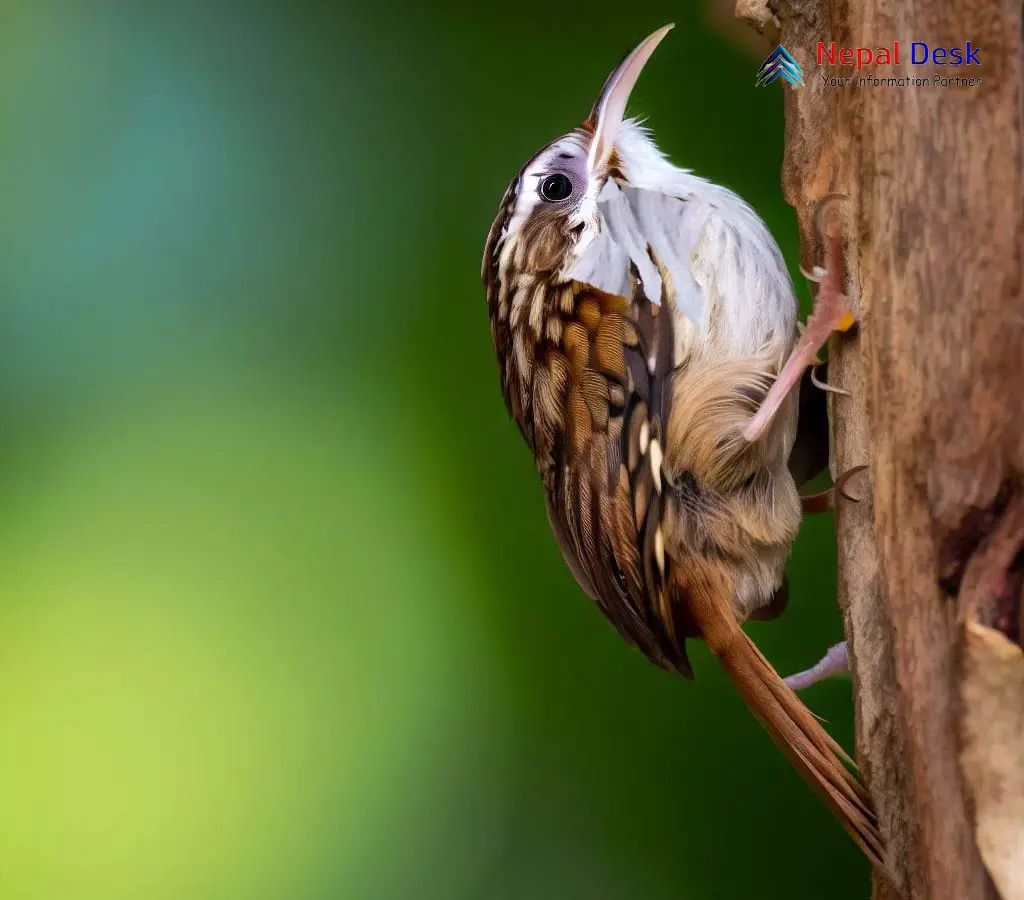This detailed close-up photograph captures a small, cool-looking bird clinging to the side of a wooden structure, likely part of a tree. The bird boasts a distinctive plumage with white feathers under its beak and a mix of black and brown spotted feathers on its back. It features a somewhat long, brownish tail and a beak that is tan or pinkish in color. While the bird doesn’t quite match a typical woodpecker's appearance, it exhibits a similar behavior by holding onto the wood. The overall setting is blurred with a green background that emphasizes the bird as the main focal point. In the upper right-hand corner, the text "Nepal Desk Your Information Partner" is visible, with 'Nepal' in red and 'Desk' in blue, indicating that the image was likely taken in Nepal. The bird’s unique pose, almost appearing as though it has four legs, adds to the intriguing nature of the image.